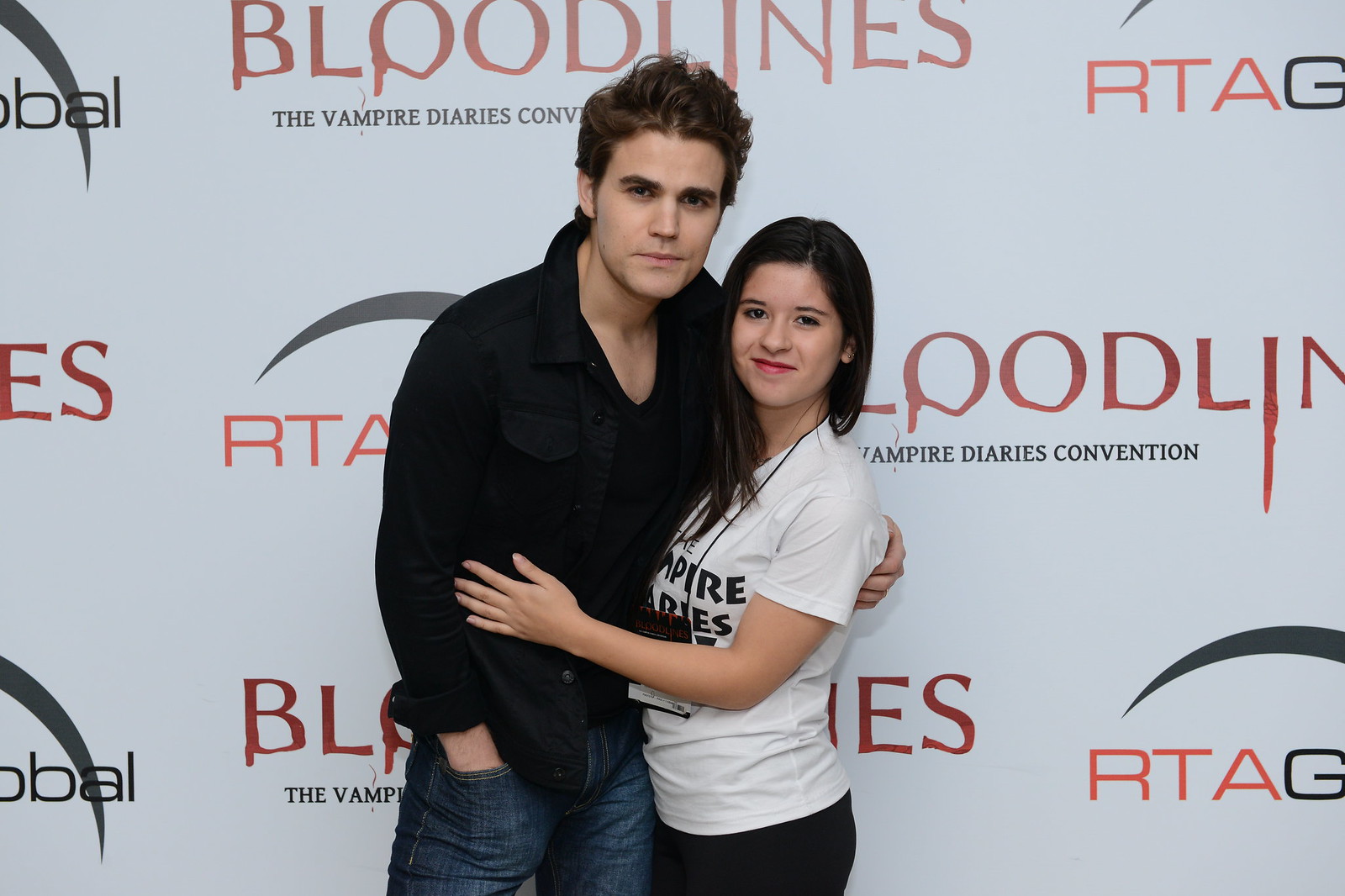A young man and woman, likely actors, are posing in front of a white wall with various inscriptions. The background features the word "Bloodlines" printed multiple times in red at the top center and elsewhere on the wall. Beneath it, in light black-gray lettering, are the words "The Vampire Diaries," partially obscured by the man. The letters "RTAG" also appear on the wall, along with a black rainbow shape above. The man stands on the left, has dark brownish hair, and is light-skinned. He is wearing a long-sleeved, black shirt that is unbuttoned to reveal a black t-shirt underneath, which has a pocket flap and is rolled up at the cuffs. His right hand is tucked into his jeans pocket, and he has his arm around the woman's shoulder. The woman, standing on the right, has dark hair draped over her shoulder, and is wearing a white short-sleeved t-shirt that also says "Vampire Diaries" and black pants. She has her left hand over the man's chest area, and they both look straight at the camera.